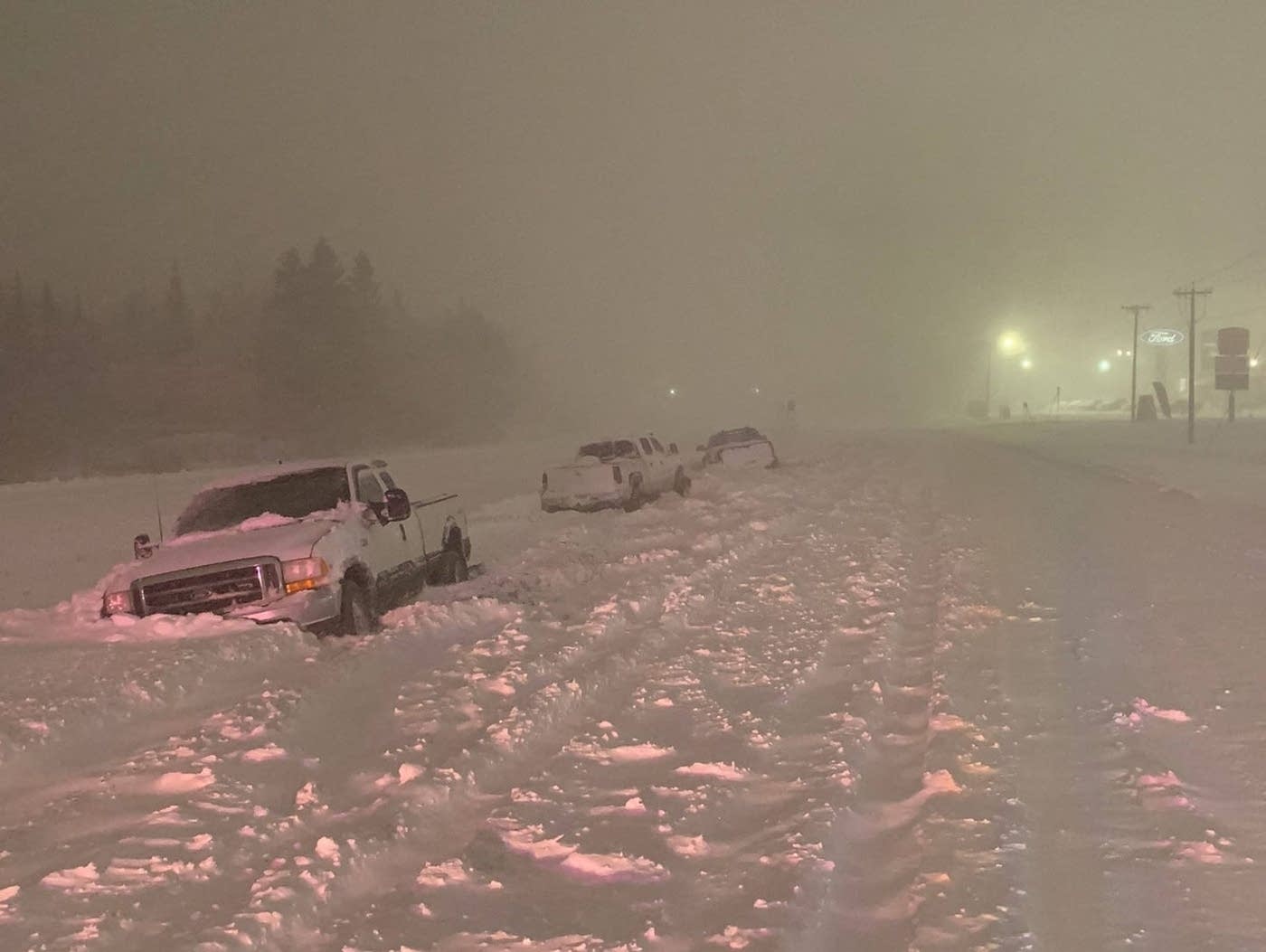This square photograph captures a wintry, snowy evening during what appears to be a snowstorm. The bottom half of the image is blanketed with multiple inches of bright white snow. Three white pickup trucks, all extended cabs, are stuck in the snow along the left side of a road. One Ford pickup, partially covered in snow, faces the camera, while another white pickup is directly behind it, showing its backside. A third truck, positioned diagonally in front of the others, has its headlights on, casting a brighter patch of light on the snow and contributing to the overall illumination. Streetlights with yellowish hues punctuate the scene, adding to the ambient glow. In the upper right, a Ford sign is visible across the road, possibly indicating a dealership or business. The sky is a murky blanket of gray, and tall pine trees frame the upper left side of the image, enhancing the wintry atmosphere.